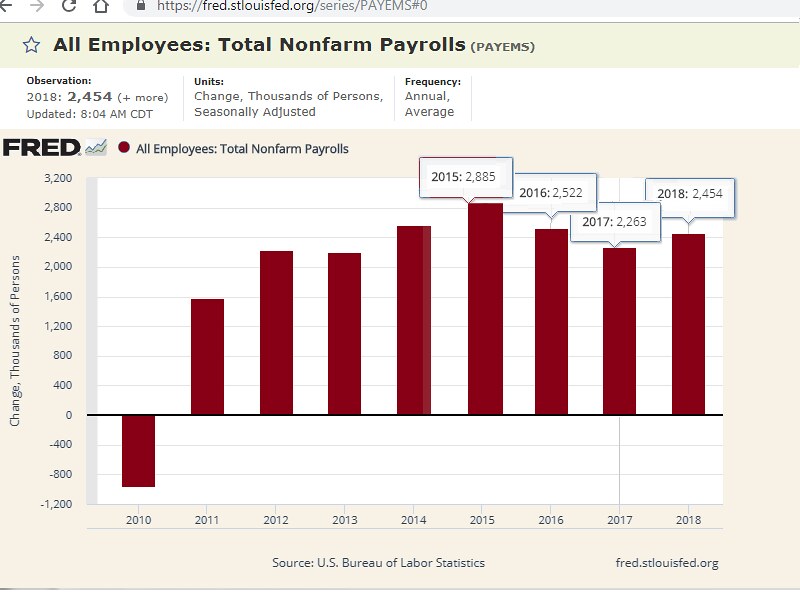The image is a detailed bar graph captured from a website, specifically from fred.stlouisfed.org/series/PAYEMS. At the top of the image, the URL and a label indicating "All Employees: Total Non-Farm Payrolls" are visible. The graph charts data from the U.S. Bureau of Labor Statistics and displays yearly changes in non-farm payrolls from 2010 to 2018. The y-axis measures changes in thousands of persons, ranging from -1,200 to 3,200, while the x-axis marks the years. The dark red bars represent annual changes, with notable fluctuations: a dip in 2010 around -1,000, a rise to approximately 1,600 in 2011, peaking near 3,200 in 2015, and varying heights through subsequent years, showing another increase in 2018. A black line denotes zero change, highlighting the positive and negative shifts in employment over the period. The graph's consistent burgundy-colored bars visually depict the national employment trend in non-farm sectors.